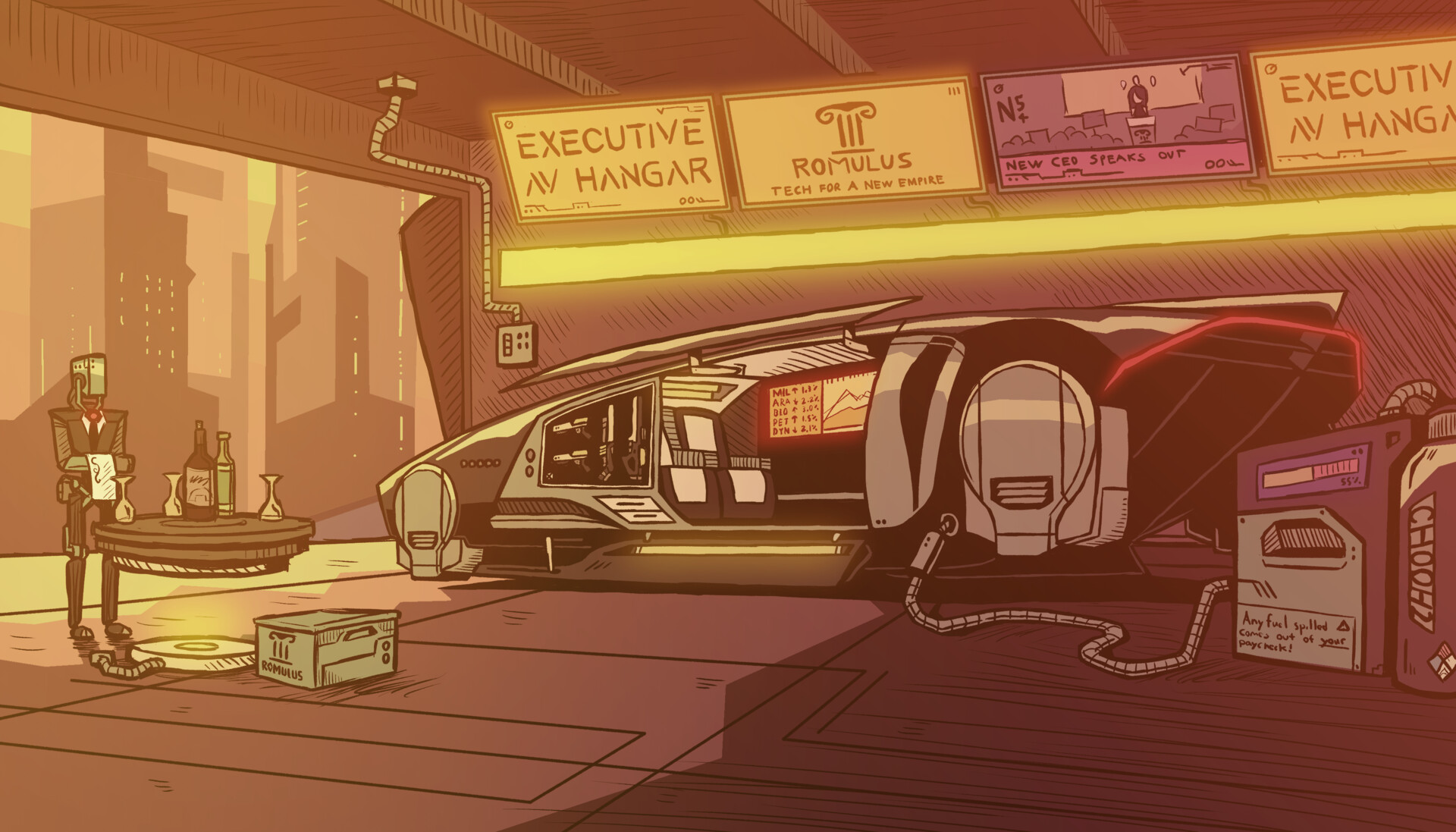The image portrays a detailed, cartoon-like, futuristic comic book-style setting within a high-tech hangar or executive space. Through an expansive window or doorway to the left, a bustling cityscape of towering skyscrapers can be seen, suggesting a sci-fi metropolis. Dominating the indoor scene is a sleek, advanced vehicle reminiscent of something from "Back to the Future," currently plugged in for charging. Prominent signs above the scene read "Executive AV Hangar" and "Romulus Tech for a New Empire," hinting at an elite, cutting-edge environment. A billboard advertises "New CEO Speaks Out," adding to the executive ambiance. Nearby, a humanoid robotic butler stands with a napkin draped over its arm, holding an elevated tray laden with champagne bottles and wine glasses, adding a touch of opulence. The overall setting feels like a luxurious, futuristic haven, blending high technology with executive sophistication.